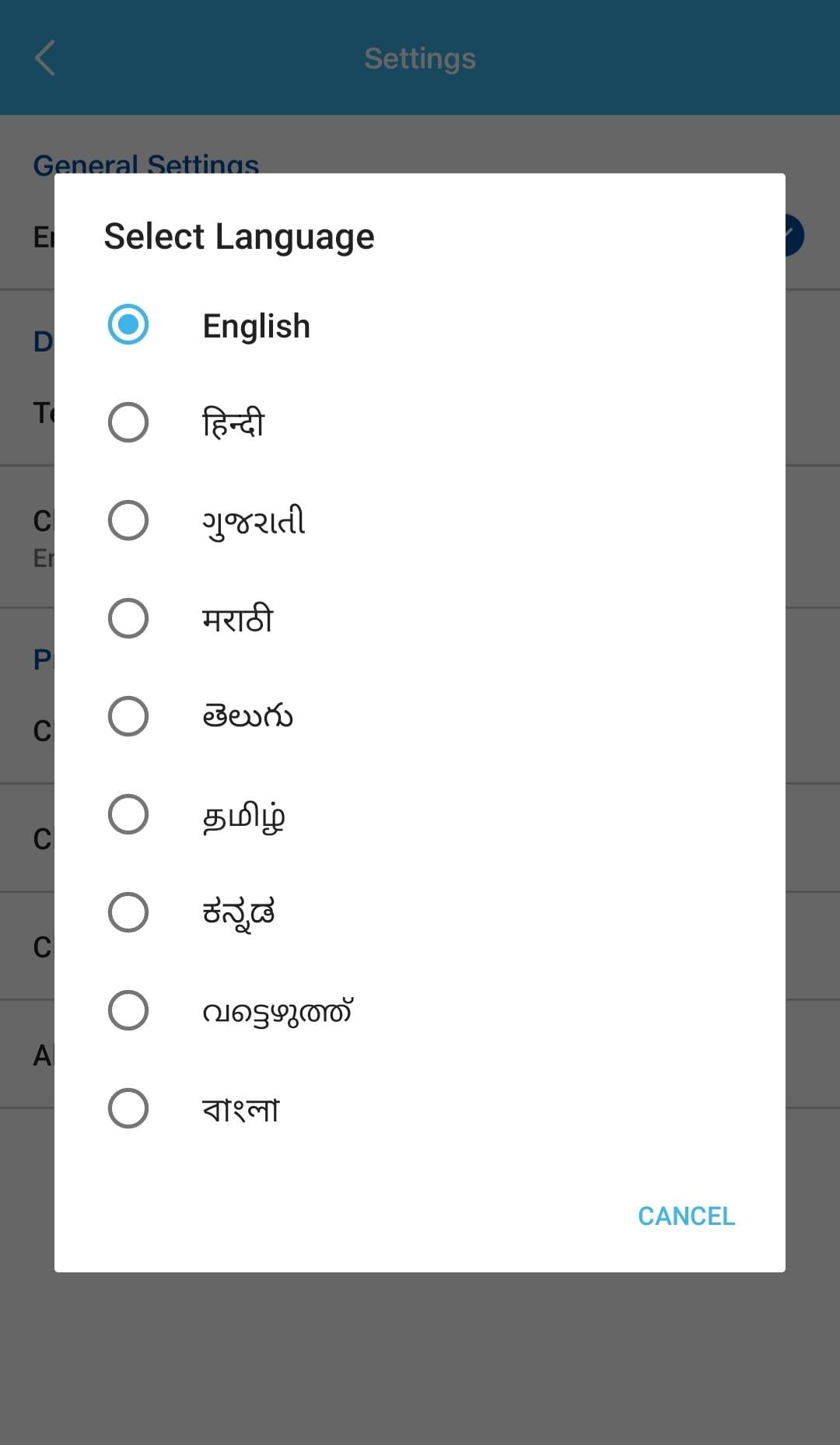In the image, we see a screenshot of a settings interface. The background features a grayed-out area, with a blue rectangle in the center displaying the word "Settings" in white text. Dominating the foreground is a pop-up window. At the top left of this pop-up, a white rectangle contains the text "Select Language," with "English" highlighted as the currently selected option. Additionally, there are eight other language choices listed beneath it.

The bottom right corner of the pop-up features a blue "Cancel" button. In the background, partially covered by the pop-up, the heading "General Settings" is visible near the top. Below this heading, only the first letters of additional sections are discernible, listed in sequence as: E, D, T, C, E, P, C, C, C, and A. The remaining area beneath these partially obscured sections appears to be white but is shaded gray due to the overlay of the pop-up window.